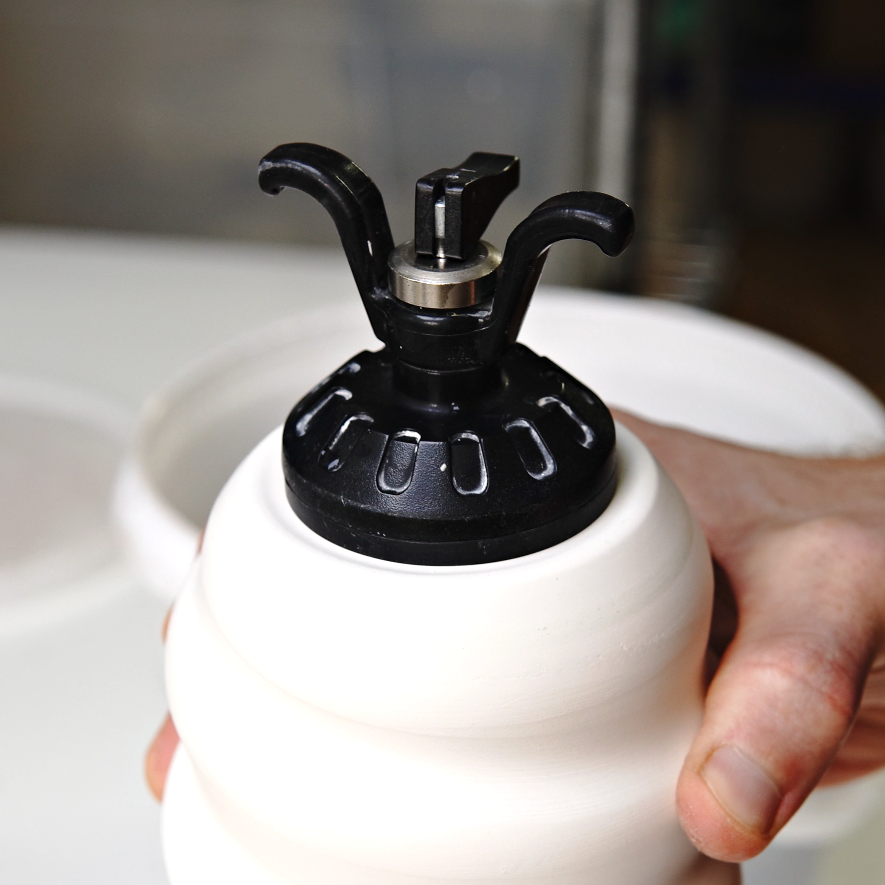This color close-up photograph captures a right hand, likely of a Caucasian male in his 20s or 30s, holding a white cylindrical object with a beehive or stacked donut-like shape. This object appears to be made of clay at the base, featuring a black metal lid with a nozzle-like fixture on top. The fixture includes a white washer and two black metal protrusions, suggesting it could be a dispenser for liquid soap or lotion, though exact identification is unclear. The hand is partially cropped, showing only the thumb and fingers grasping the object. The background is out-of-focus with white and black blurry areas, potentially indicating a white tabletop or sink and a darker patch in the upper right corner.